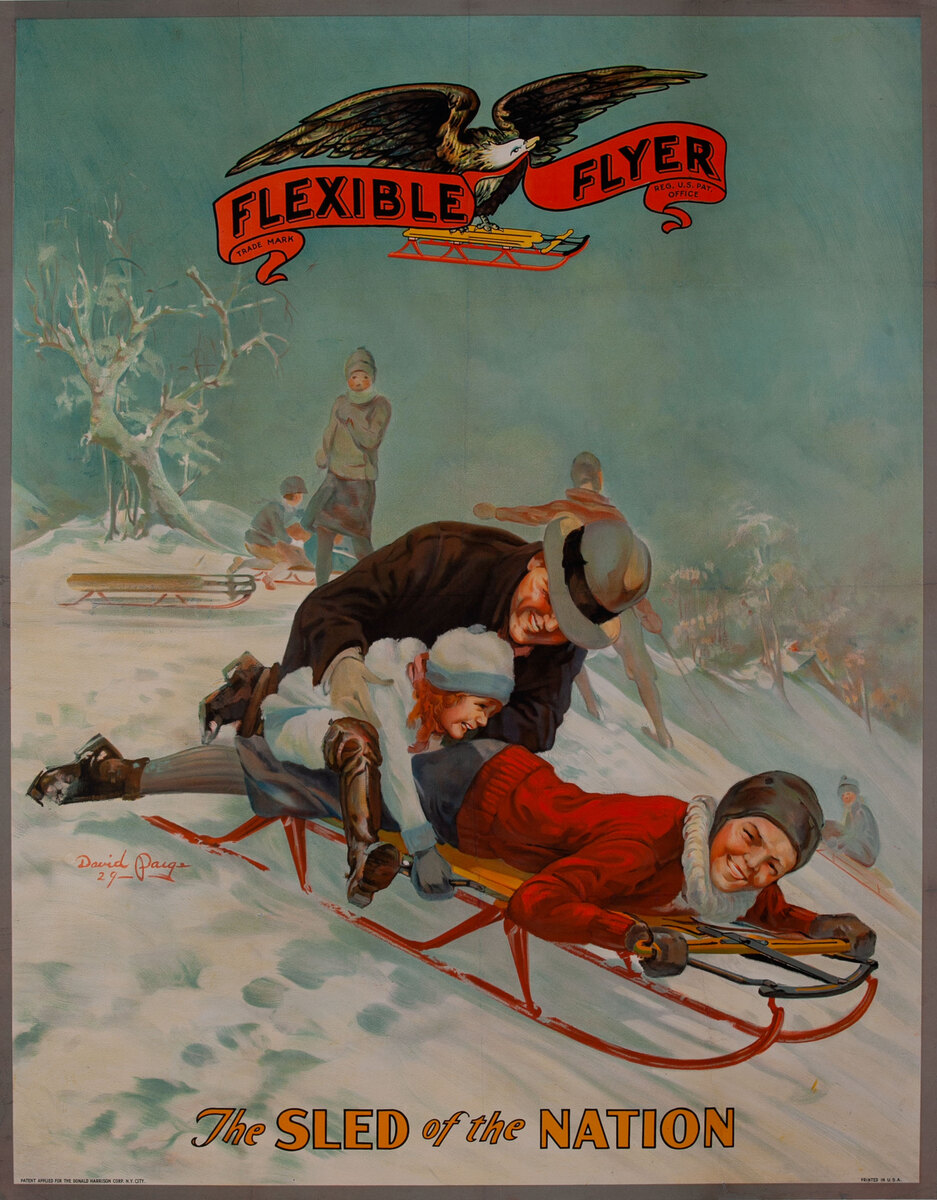The image depicts a vintage advertisement from the 1940s or 1950s for the Flexible Flyer, known as "The Sled of the Nation." Rendered in a classic, stylized manner reminiscent of Norman Rockwell's work, it showcases a family engaged in a joyful sledding scene on a snowy hill. Central to the image is a father placing his young daughter onto the back of her brother, both dressed warmly in winter attire, aboard a red-and-blue wooden sleigh with red metal runners. Surrounding them in the snowy landscape are other children and adults enjoying sledding activities, some watching and others preparing to descend the slope. An iced-over tree is visible to the left, adding to the wintry atmosphere. At the top of the image, an eagle holding a banner with "Flexible Flyer" stands on a sled, while the bottom of the image features the slogan "The Sled of the Nation" in orange letters. The background is a greenish-blue hue, evoking distant trees and enhancing the nostalgic charm of the scene.